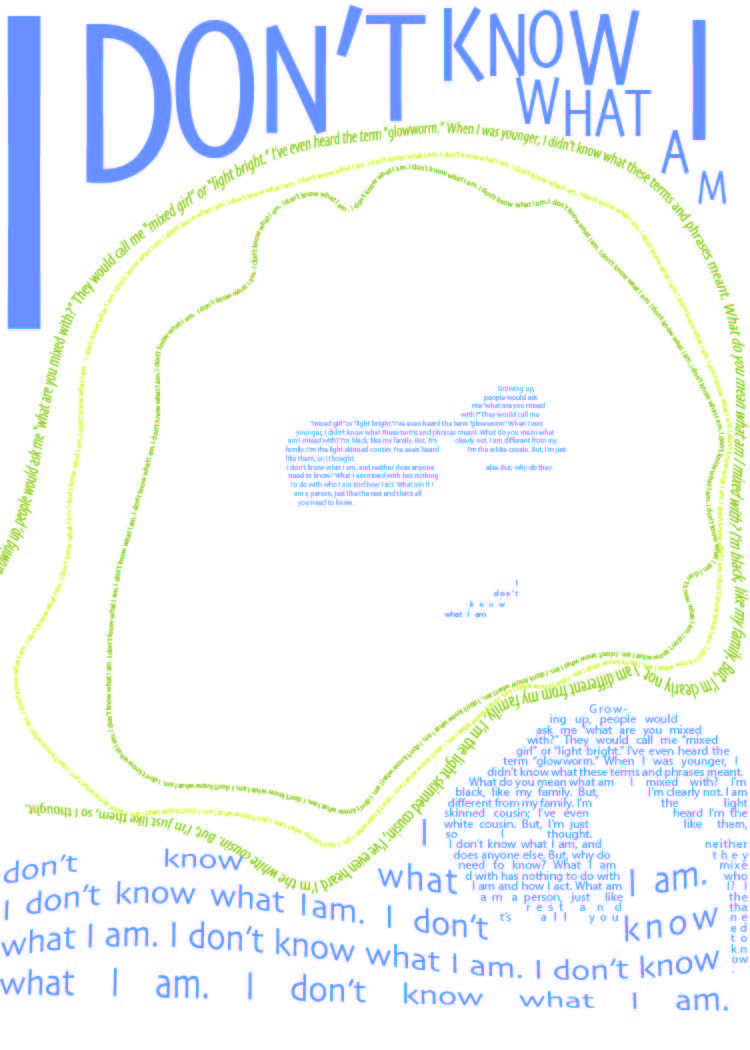The image depicts a digital art piece designed as an abstract representation of a face composed entirely of text elements. Dominating the artwork, large blue letters spell out "I don't know what I am" across the top with a distinctive spacing that makes the text appear as though it is disintegrating. The face itself is outlined using curving, psychedelic, greenish-yellow text forming an oval shape with bumps and valleys. Within this outline, blocks of blue text simulate eyes, and beneath them, another block addresses the mouth area, spelling "I don't know who I am." Below this facial formation, a dense wall of blue text shapes the likeness of shoulders and a chest region, repetitively incorporating the phrase "I don't know what I am." Additional text at the bottom narrates a personal reflection on mixed-race identity, with phrases recalling childhood experiences and the confusion about their ethnic background: "growing up people would ask me, what are you mixed with...? I'm black like my family but I'm clearly not." The piece, while rich in emotive language and form, features large areas of unused space, adding to its introspective and somewhat unfinished visual narrative.